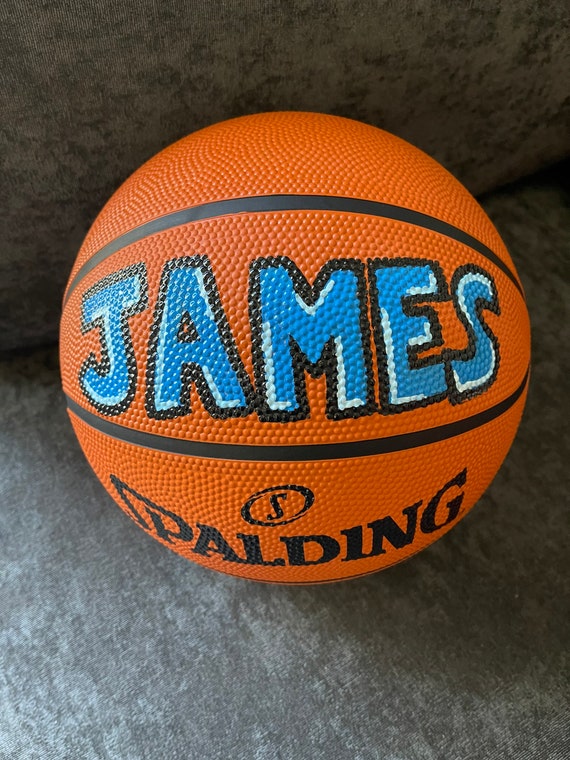The image features a standard orange basketball resting on a gray, marbleized surface that resembles stone but might also be fabric, such as a couch. The basketball, marked with the characteristic black lines for grip, prominently displays the brand "Spalding" along the bottom, accompanied by the brand's oval logo with the letter 'S' in the middle. Above the brand name, the word "James" is printed in large, capital letters. The name "James" is uniquely detailed, with each letter outlined in black and filled with dark blue, highlighted with lighter blue on parts of the edges, giving a reflective or shadowed effect. The basketball is centrally placed in the photo, drawing attention to both its distinct markings and the textured surface beneath it.